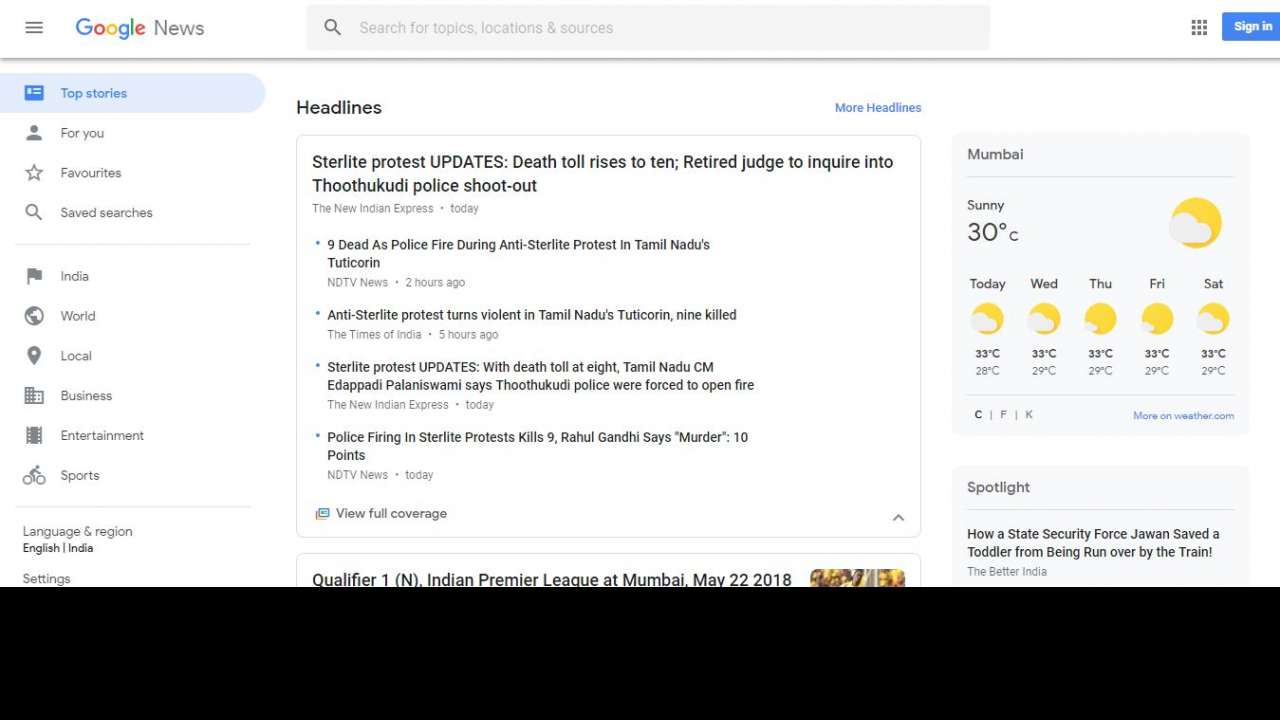Certainly! Here's a detailed and cleaned-up caption for the image described:

---

**Description: Google News Webpage Interface**

The image depicts the interface of a Google News webpage. In the upper left-hand corner, there are three horizontal black lines stacked vertically, indicating a menu icon. To the right of this icon, the Google logo is prominently displayed, with the letters "G" in blue, "O" in red, the second "O" in yellow, the second "G" in blue, the "L" in green, and the "E" in red.

To the right of the Google logo, the word "News" is written in black. Centered at the top of the page is a gray search bar with a magnifying glass icon on the left. Within the search bar, placeholder text reads, "Search for topics, locations & sources."

On the right side of the search bar is a square icon composed of nine smaller squares arranged in a 3x3 grid, symbolizing Google apps. Next to this icon, a blue rectangular button reads "Sign in" in white text.

Beneath the top section, in the upper-left corner, the section "Top Stories" is highlighted in blue. Below this, there is an icon of a person (depicting head and shoulders), labeled "For you." Subsequently, a star icon with the label "Favorites" follows, then an icon of a magnifying glass next to the label "Saved Searches." 

Continuing down the left-hand side, there is a flag icon labeled "India", a globe icon labeled "World", a map pin icon labeled "Local", and an icon of two buildings labeled "Business." Further down, there is a filmstrip icon labeled "Entertainment", followed by a stick figure on a bicycle icon labeled "Sports." At the bottom of this column, there is text reading "Language & Region", "English", followed by "India", and "Settings."

In the central column of the page, the headline "Sterlite Protest Updates: Death Toll Rises to 10, Retired Judge to Inquire into Thoothukudi Police Shootout" is listed under "Headlines." This section is attributed to "The New Indian Express" and dated today. Bullet points include updates such as:
- "Nine dead as police fire during anti-Sterlite protest in Tamil Nadu's Tuticorin."
- "Anti-Sterlite protest turns violent in Tamil Nadu's Tuticorin; nine killed."
- "Police firing in Sterlite protest kills nine; Rahul Gandhi calls it 'murder'."

An option to "View Full Coverage" is available. Below, there is a sports update for the "Indian Premier League Qualifier 1" held in Mumbai on May 22, 2018.

On the far-right column, the weather for Mumbai is displayed. The top section reads "Mumbai," with a sunny icon and the temperature "30°C." The weather forecast for the week follows, listing daily highs of 33°C and lows varying between 28°C and 29°C for Tuesday through Saturday.

---

This caption provides a thorough description of the various elements and layout of the Google News webpage as observed in the image.